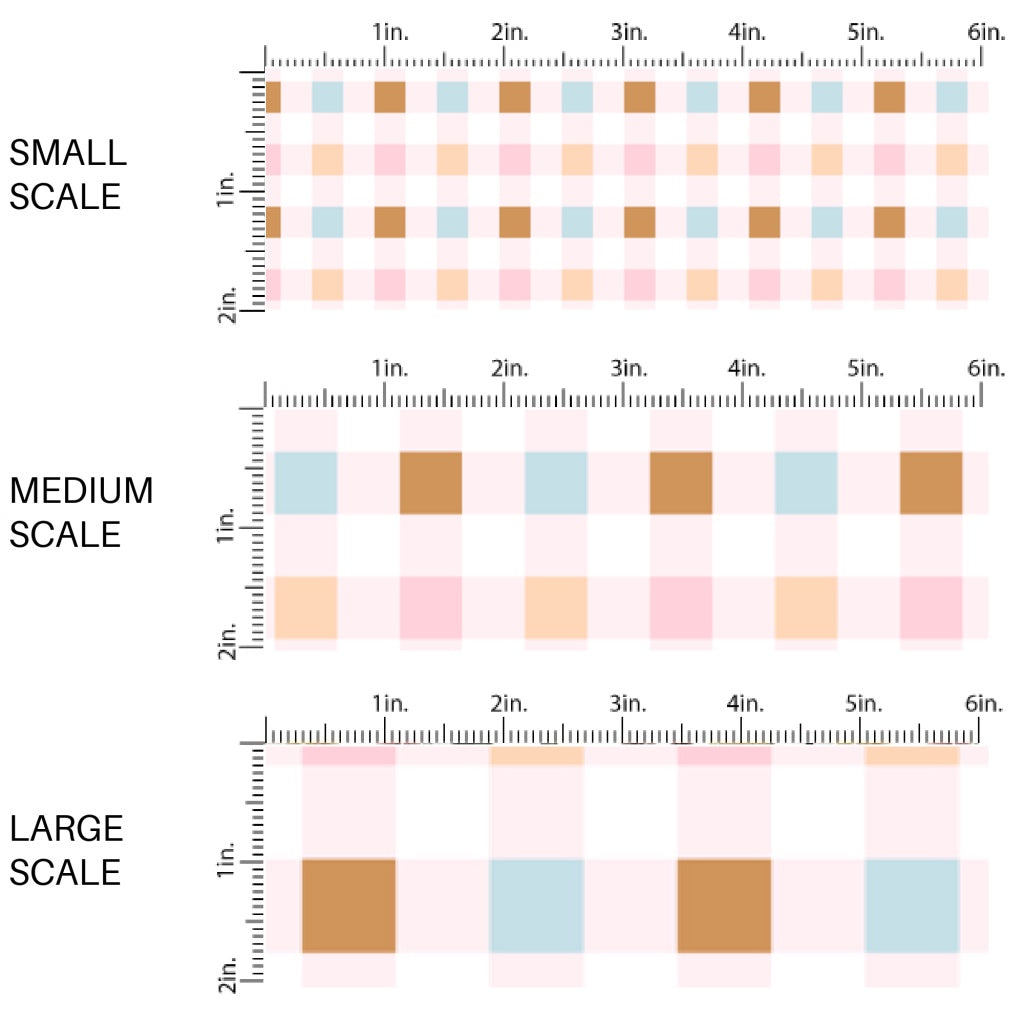The image depicts three separate illustrations labeled "small scale," "medium scale," and "large scale," arranged from top to bottom. Each illustration features a grid-like pattern with a roller scale on the top and left sides. The top roller measures up to 6 inches, marked at 1-inch intervals, while the left roller is marked at 1-inch and 2-inch intervals. 

In all three illustrations, a checkerboard pattern is visible, consisting of squares in multiple colors including light blue, light brown, light pink, light orange, beige, and white. These colors are consistent across the different scales. 

The "small scale" has densely packed squares with each measuring about an eighth of an inch. The "medium scale" features larger squares, approximately one-quarter to one-half inch each. Finally, the "large scale" showcases the largest squares, nearly half an inch each. The illustrations also highlight a repeated alternating pattern of light and dark shades, creating a cohesive visual representation across varying scales.